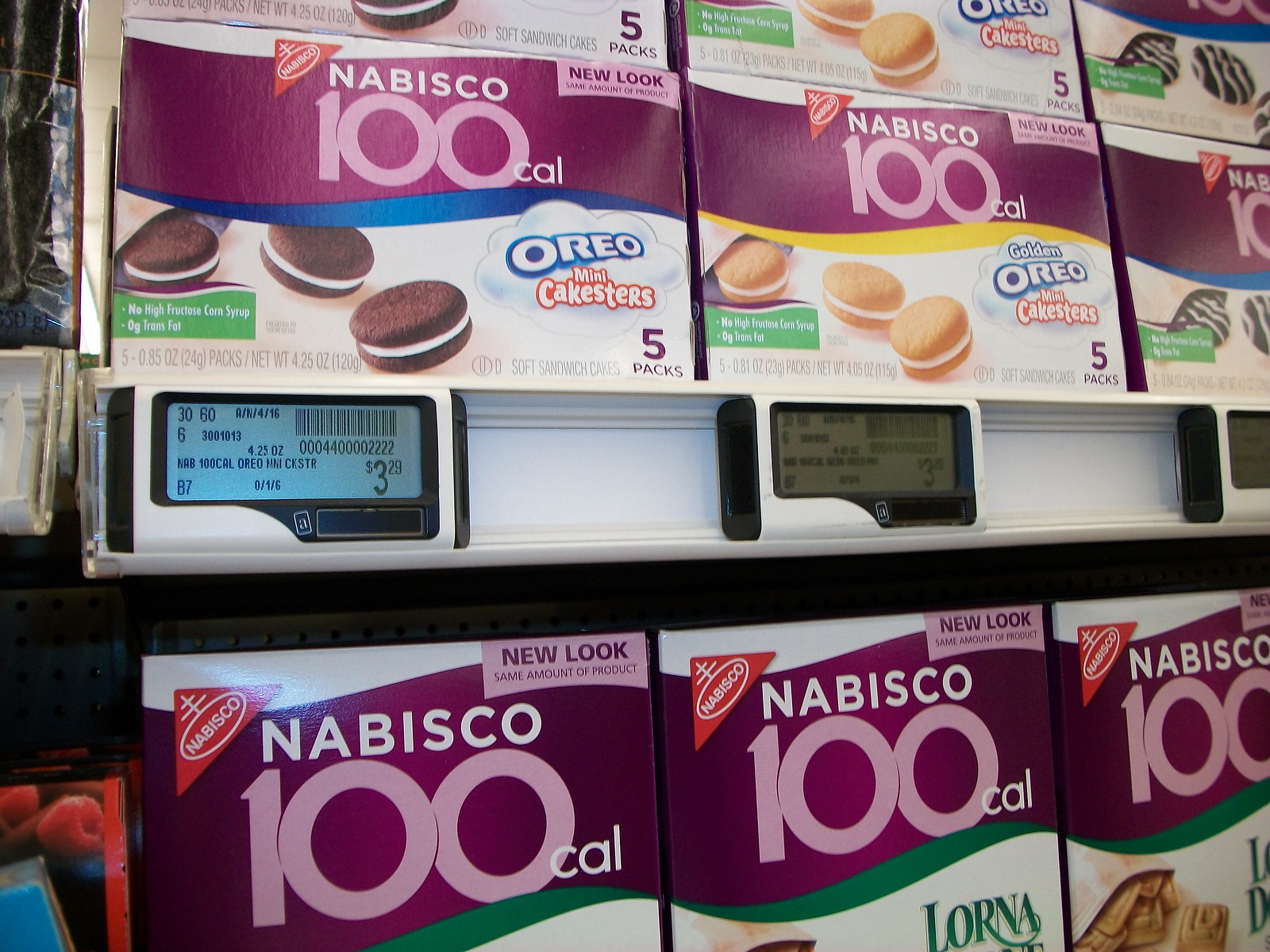This indoor color photograph, taken in a grocery store, provides a close-up view of a shelf display featuring Nabisco brand products, specifically Oreo Mini Cakesters. The focus of the image is on digital price tags that clearly display prices, with one showing $3.29. The central shelf is lined with white boxes featuring purple labels stating "Nabisco 100 calorie" and "Oreo Mini Cakesters" mainly in the lower right corner of the packaging. Above and below this main shelf, additional rows of these boxes are visible, with the triangular Nabisco logo prominently placed in the upper left corner. The digital tags underneath each product include barcodes and numerical prices. The design of the packaging includes a slightly curved dark burgundy banner with a thinner, colorful banner underneath, which varies in color among blue, yellow, and green. The photograph captures a neat arrangement of the products, emphasizing the organized display within the grocery store setting.